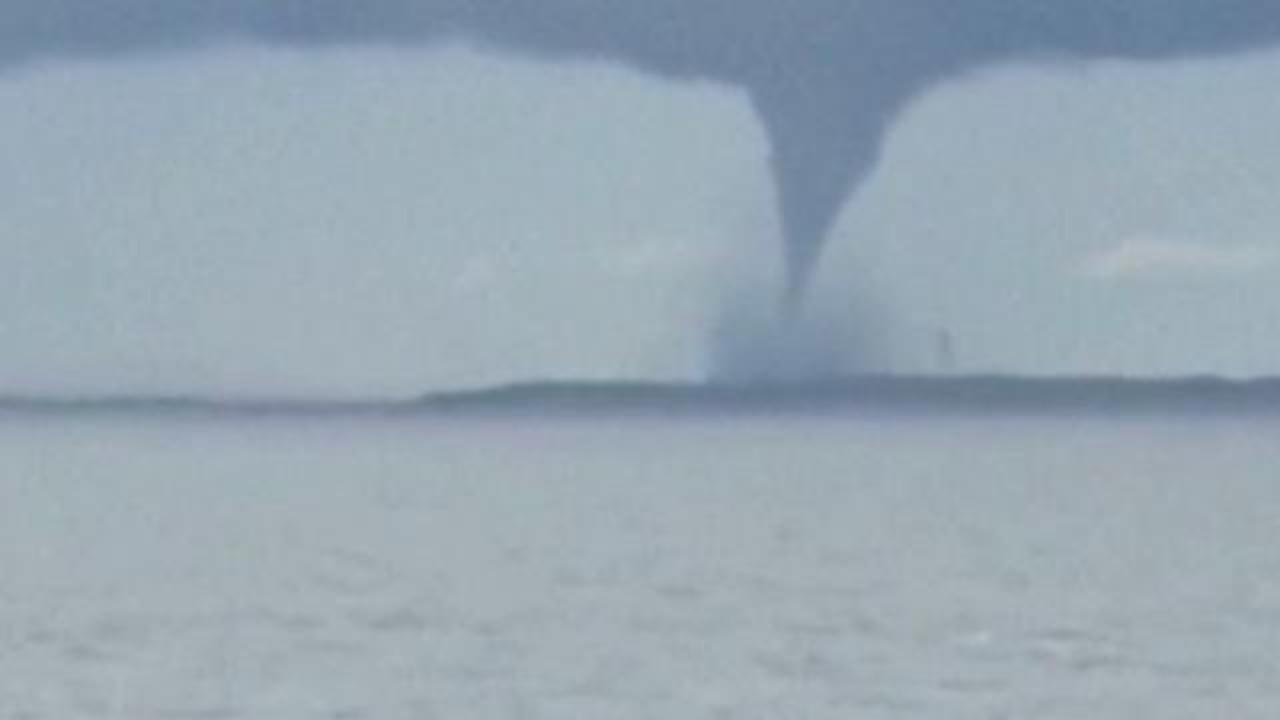The photograph captures an ominous nautical scene featuring a dramatic waterspout, also commonly referred to as a tornado over water. The image, which spans more in width than height, shows a large, steel gray body of water occupying the lower half, devoid of any boats, people, or vehicles. The horizon, slightly right of center, reveals a dark gray waterspout rising from the sea, surrounded by misty debris at its base. The sky above is filled with various shades of blue-gray and steel gray clouds, contributing to the muted, almost monochromatic color palette of the image. Despite its aged and slightly out-of-focus appearance, the photograph clearly depicts the vortex stretching from the darkened horizon up to the top of the frame. The scene is brightly lit, enhancing the stark contrast between the tumultuous waterspout and the somber, gray surroundings.